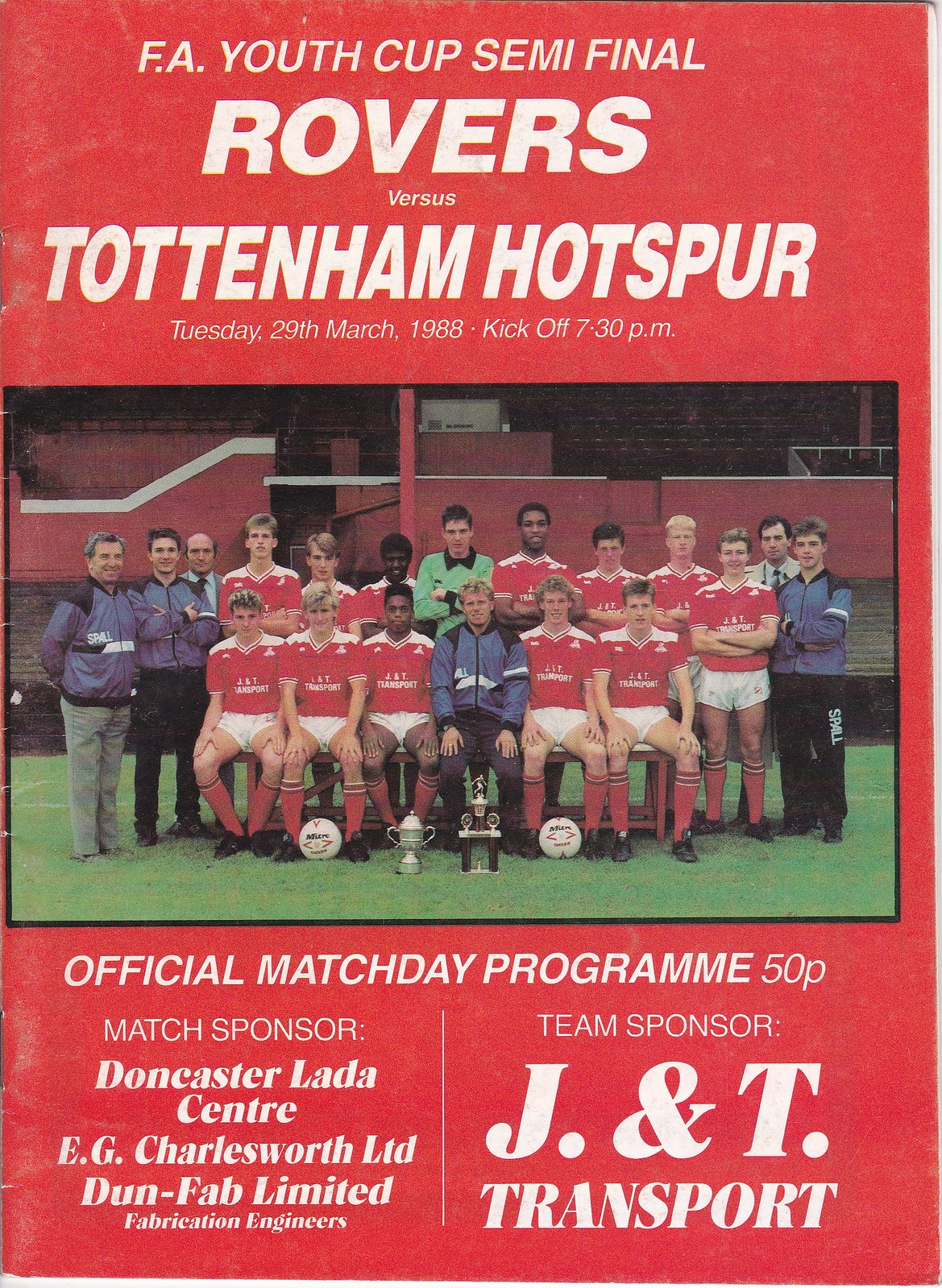The image depicts a vintage-styled flyer for the F.A. Youth Cup Semi-Final, prominently featuring a photograph and set against an entirely red background. At the very top, bold white text reads "F.A. Youth Cup Semi-Final," followed by "Rovers" in large letters, "Versus" in smaller font, and "Tottenham Hotspur" again in a large font. Details of the event are listed beneath: "Tuesday, 29th March 1988, Kickoff 7:30 PM." Centrally placed is a rectangular, landscape-oriented photograph of the participating team members, seated in a stadium setting with their coaches and managers. The team is dressed in red and white jerseys, white shorts, tall red and white socks, and black cleats. One player, presumably the goalie, stands out in a green outfit with a black collar. In front of the team are two trophies and two soccer balls. Below the photograph, text reads: "Official Match Day Program, 50p." Flanking this text, the left side lists the match sponsors, "Doncaster Lada Center, EG Charlesworth Limited, Dunfab Limited Fabrication Engineers," while the right side acknowledges the team sponsor, "J&T Transport."